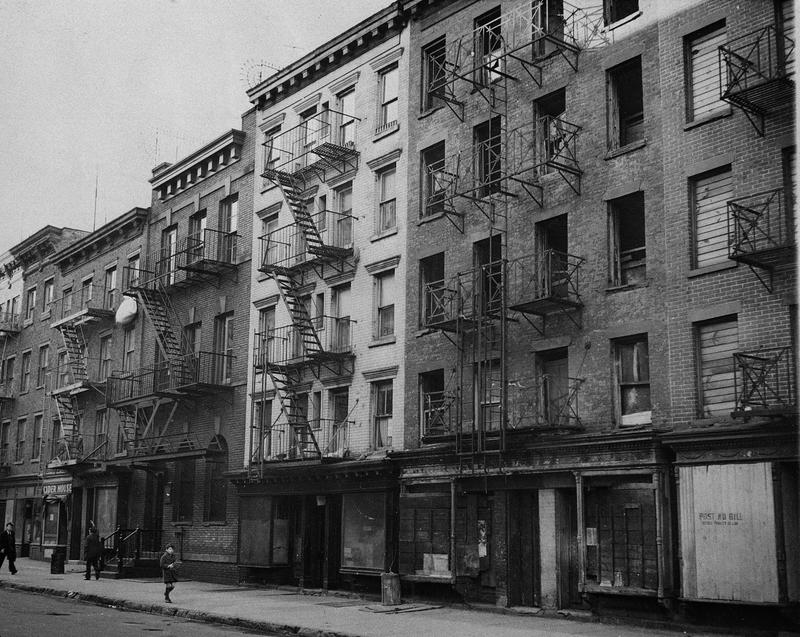This black and white photograph captures a row of old-fashioned, five-story apartment buildings, likely brownstones, in a large city from perhaps the 1920s. The buildings are constructed of brick and feature intricate fire escapes scaling their facades. Distinctively, the far right building has a row of windows that are boarded up, including the bottom one. The image includes a glimpse of the street at the bottom left corner, where a sidewalk traverses in front of the buildings. On this sidewalk, three men can be seen, spaced apart and walking in different directions, some dressed in suits and ties. The sky is partially visible in the top left corner, completing the scene.